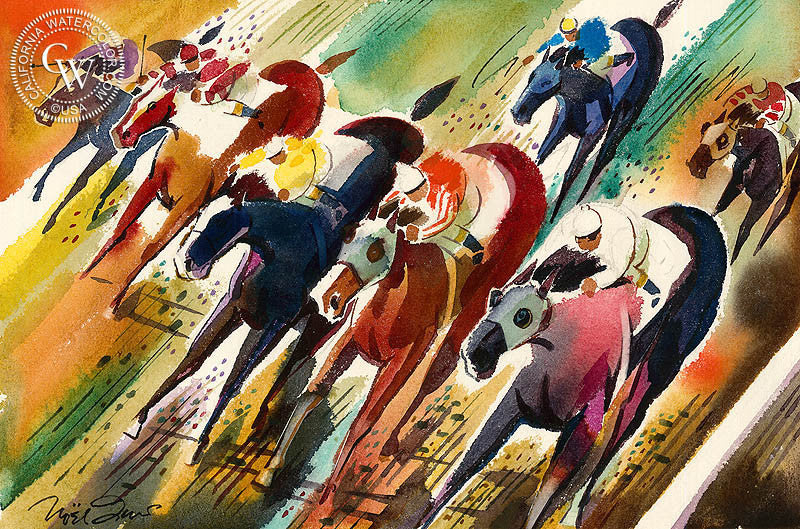This wide rectangular watercolor painting vividly captures the intensity of a horse race, showcasing a dynamic composition of horses and jockeys racing diagonally across the frame. The largest and closest horse, positioned at the bottom right corner, charges towards the bottom left. This horse features a striking gradient from pink at the front to blue at the back and wears a green mask. Mounted by a jockey dressed in white and green with a white cap, this horse stands out prominently. Just behind it, under the top right corner, is another horse, and to their left, spanning up to the top left corner, are four other horses, each with unique masks and colors, creating a vibrant and chaotic scene. The race track itself is a dazzling array of rainbow watercolors that mirror the motion of the horses, enhancing the feeling of speed and movement. This painting, possibly stamped with "California watercolor.com, USA," and marked with a signature at the bottom left, conveys a sense of frantic motion and competition, with the colors and brushstrokes giving an impression of rapid movement. All jockeys are depicted faceless, emphasizing the anonymous, universal intensity of the race.